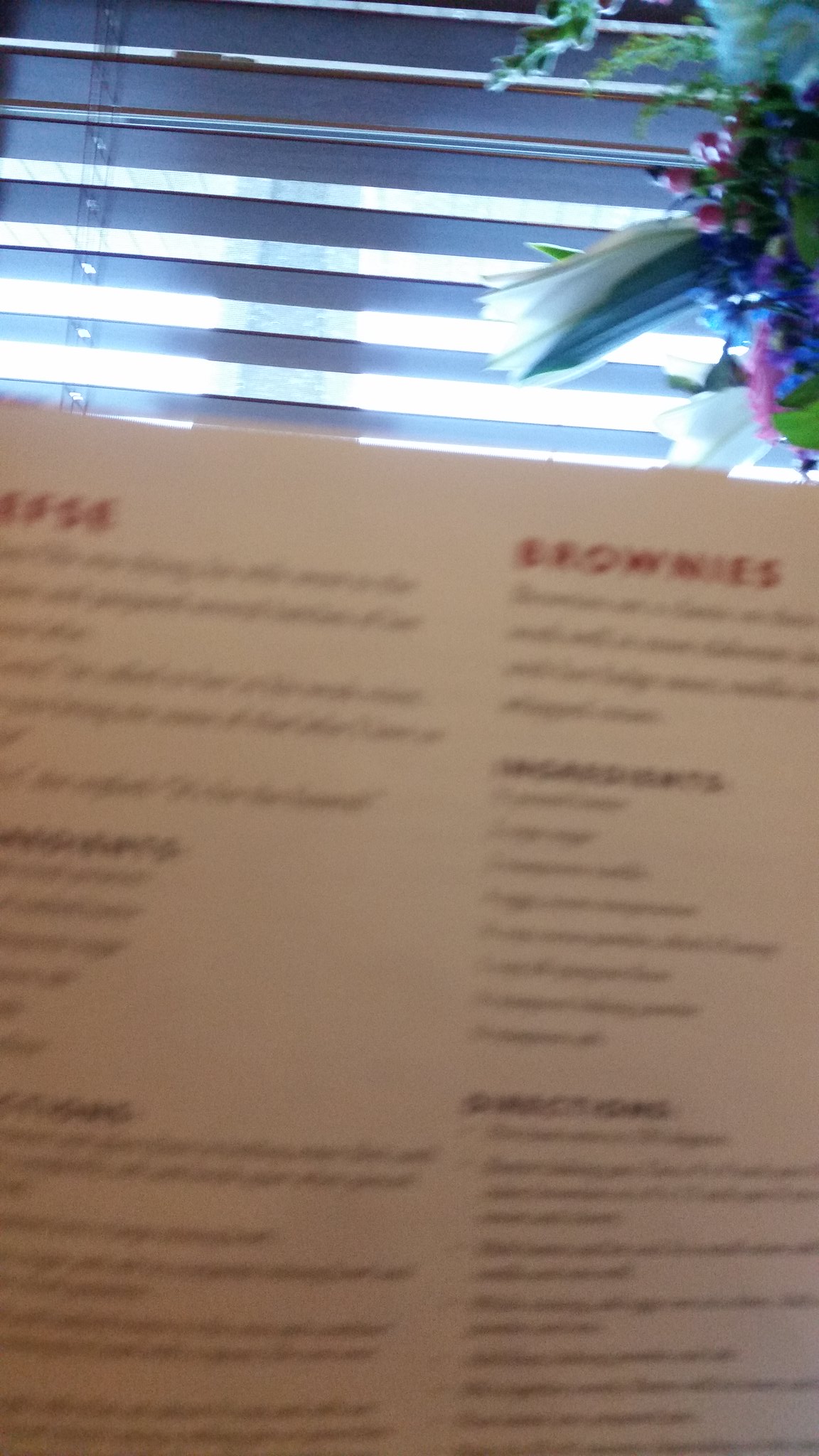This photograph is a vertically oriented, out-of-focus image capturing the scene in what appears to be a restaurant or diner. The bottom two-thirds of the image shows a blurry menu or cookbook page, with a large header in red that reads "Brownies," followed by bold black text detailing ingredients and directions. The rest of the text on the menu remains indistinct due to the blurriness. The top third of the photograph features a window with brown, louvered shades in the open position, allowing bright, white light to flood in from outside, where some hedges or trees are faintly visible. In the upper right corner, there is a floral arrangement in various colors, including pinks, purples, whites, and greens. The ceiling of the building includes visible infrastructure and lights, hinting at a spacious, possibly metallic design. Overall, the image combines elements of the menu, the restaurant’s interior, and a glimpse of the exterior setting, creating a layered, albeit blurry, snapshot of the moment.